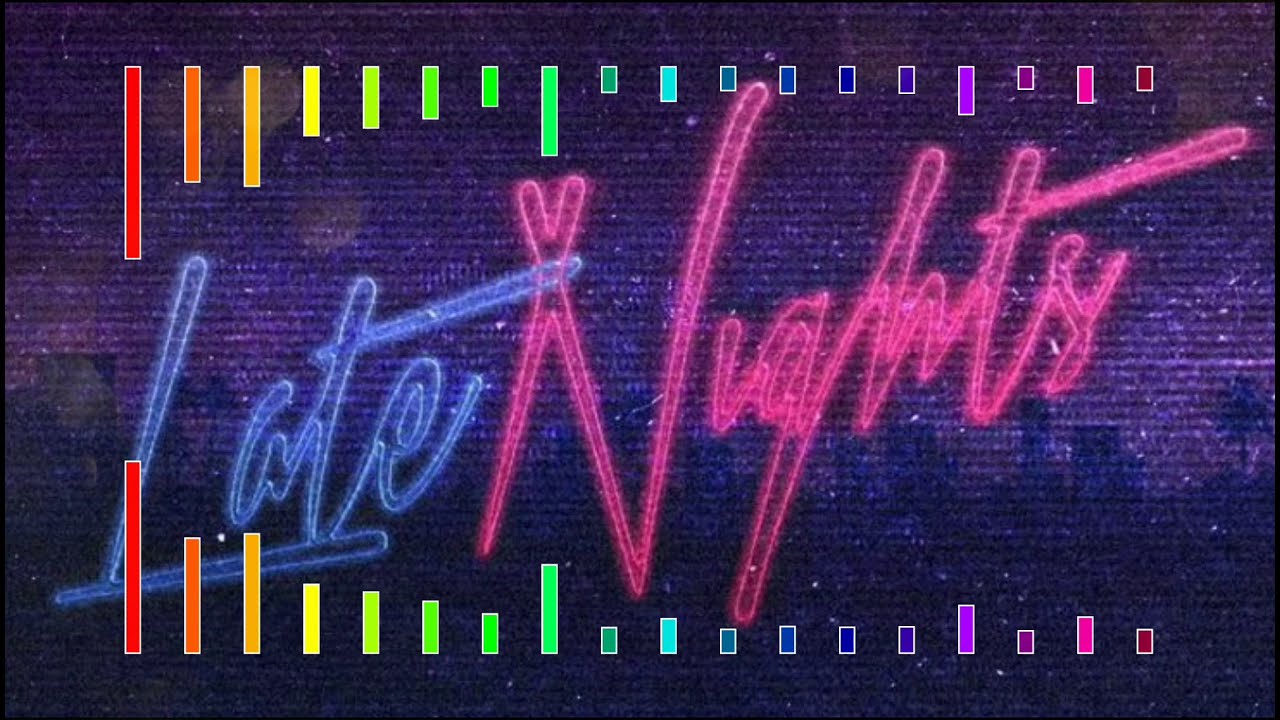The image features a digitally created label set against a background resembling old, pixelated brick in shades of blue and purple. The centerpiece phrase "Late Nights" is prominently displayed in a diagonal script that starts at the lower left and extends to the upper right. "Late" is written in blue cursive, while "Nights" is in a reddish-pink, both appearing to be illuminated. The background subtly incorporates a faint city skyline along the bottom half, adding an urban feel.

Above and below the text are thin vertical bars in a gradient of rainbow hues, forming a visually striking frame. These bars start with shades of red and orange on the left and transition through yellows, greens, blues, purples, and finally back to deep red and burgundy. The overall effect is a vibrant, colorful, and slightly worn banner that looks like a cross between a city art piece and a digital creation.